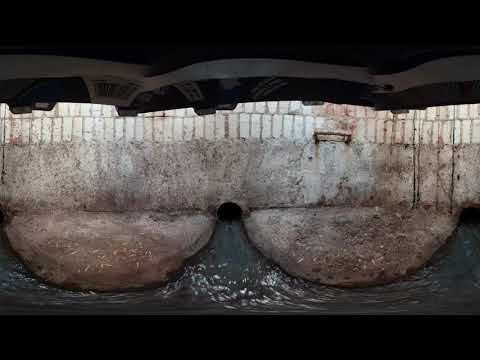The image features a detailed, horizontal cement structure at its center, adorned with a pattern of tiny rectangular shapes on its top surface. At the bottom middle of this cement block, a circular hole is visible, from which green-colored water is either flowing out or into. Flanking the hole on both sides are semi-circle cement formations. The setting appears to be a sewer system, corroborated by an additional small hole on the right side of the image and dark blue water depicted at the base, indicating water flow from the mentioned holes. In the backdrop above the cement structure, there's a stark white line, possibly a ceiling or canopy, framed by a dark border at both the top and bottom of the image. Vertical black lines also cut across the structure, adding further texture and contrast.